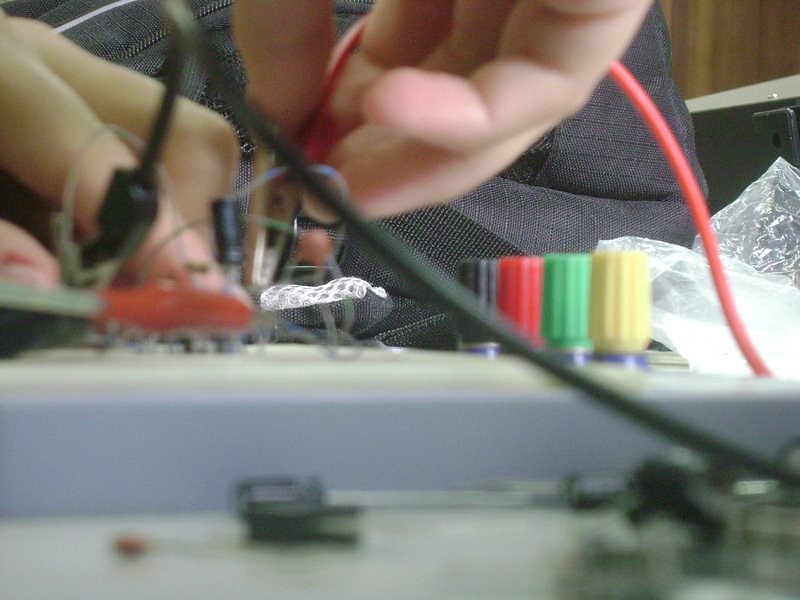The photograph captures a meticulous close-up of a pair of hands diligently working on an electronic assembly. The image, taken from a low angle as if the camera is sitting on the table, centers on the hands holding electrical wires with clamps. These hands are engaged with a rectangular control panel featuring an array of colored buttons or knobs: yellow, green, red, and black. Surrounding the main control panel are an assortment of wires, predominantly red and black, intertwining in various directions. Additional tools and small components lie scattered in front of the control panel on the table, suggesting an intricate ongoing project. The image vividly conveys a scene of focused craftsmanship and detailed electronic assembly.